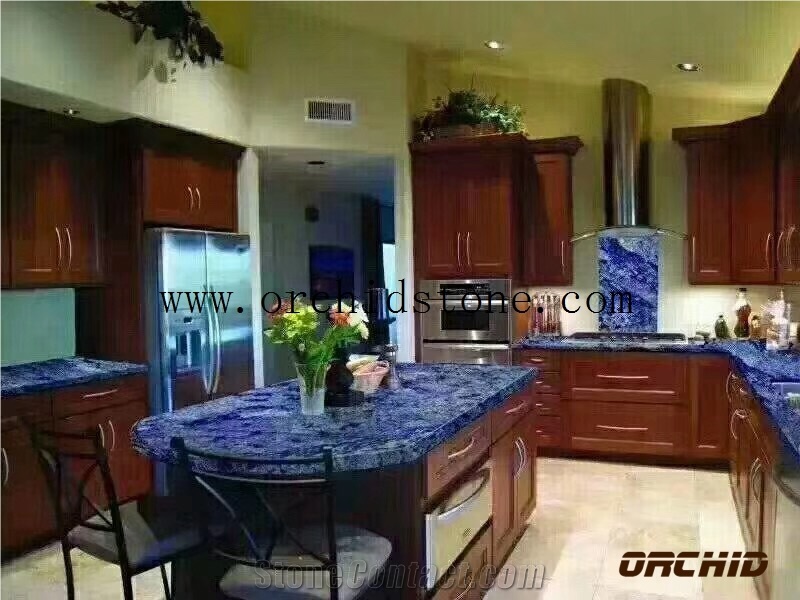The image showcases a somewhat outdated yet captivating kitchen design featuring prominently vivid blue stone countertops and backsplash made of a striking quartz or granite. Central to the kitchen is a large blue island surrounded by two black metal stools with gray cushions. The cabinetry, both on the island and lining the periphery, is a dark wood with sleek silver handles, contrasting with the stainless steel appliances that include a refrigerator to the left, a stove centrally located, and a sink on the right side. The floor is adorned with cream-colored tiles, while the walls are a beige hue that transitions to a yellowish tint towards the ceiling. Adding to the visual interest, a cylindrical silver ventilation system is positioned above the stove. While the image quality is low, reminiscent of early 2000s digital photography, it highlights the vibrant blue stone that appears almost photoshopped in its intensity. The image, an advertisement from www.orchidstone.com, features prominent black text of the website's address in the center, with "orchid" embossed in brown font crossed out at the bottom right corner and an additional watermark from stonecontact.com.